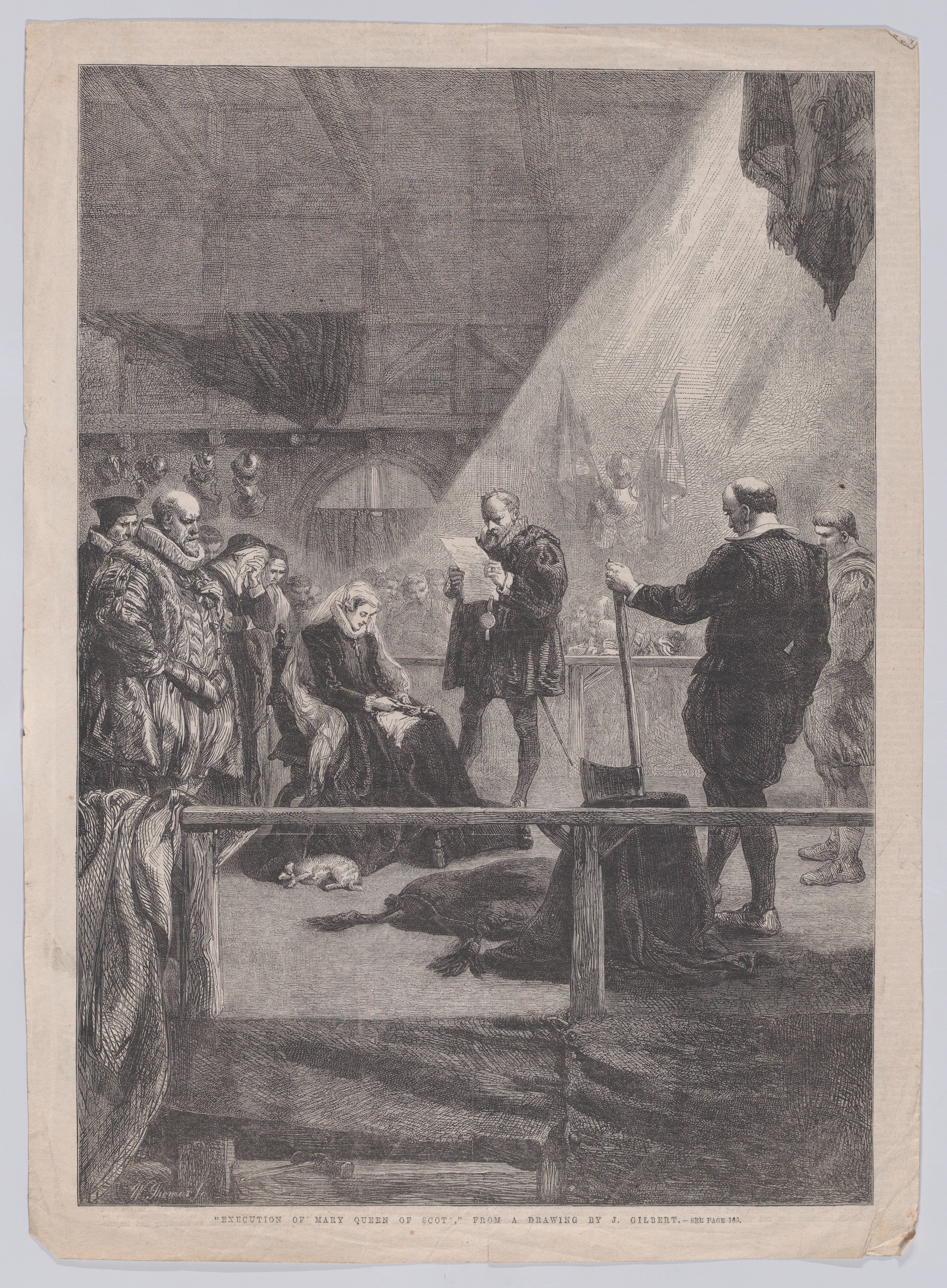This black-and-white photo captures a detailed vintage pen-and-ink illustration from a book, set against a gray background. The illustration, titled "Execution of Mary, Queen of Scots" by J. Gilbert, depicts the somber scene of Mary sitting slumped in a chair, dressed in a long, dark, flowing gown, with her head bowed in sorrow. At her feet, a cat lies asleep, adding to the poignant atmosphere. A man dressed in a short, billowy robe and tights stands before her, reading aloud from a long sheet of paper. Surrounding Mary are several onlookers in medieval, regal clothing, all sharing a posture of grief or shame with heads bowed. In the right corner, an executioner stands by with an axe resting on a tree stump, poised for the inevitable. The room itself features wooden walls and an arched ceiling, with a closed, arched doorway and sunlight streaming in from the upper right corner, subtly highlighting the gravity of the moment.